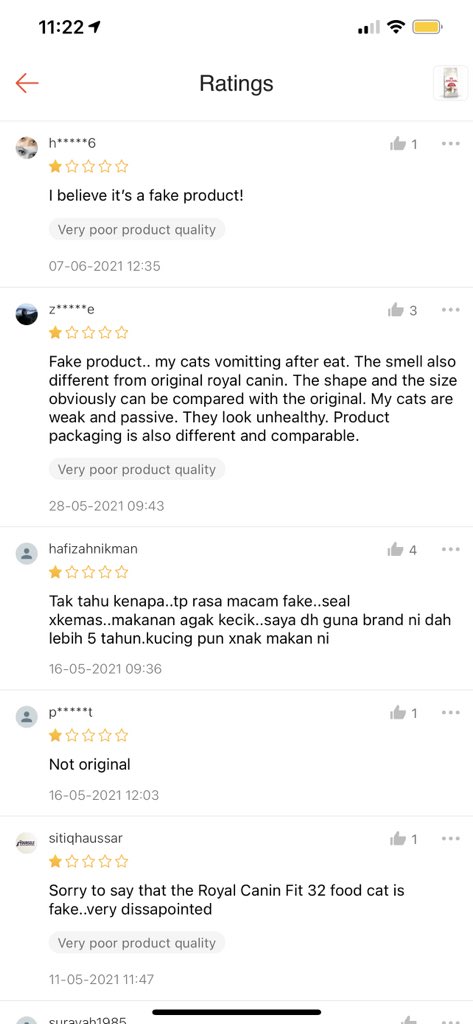The image showcases a cell phone screen against a white background. In the top left corner, it displays the time "11:22." The top right corner features icons for cellular signal, wireless connection, and battery status. Below these icons, the screen header reads "Ratings." The image then presents several product reviews, each accompanied by a small, indistinct user icon.

The first review, submitted by a user identified as "H*****6" (with part of the username blurred out), includes a thumbs-up icon with the number "1." This user rated the product 1 out of 5 stars and titled their review, "I believe it's a fake product." They express dissatisfaction, noting "Very poor product quality."

The second review is from a user named "Z*****E," who also awarded the product 1 star. Next to their review is a thumbs-up icon with the number "3." The review states: "Fake product. My cat's vomiting after eat. The smell also different from original Royal Canin. The shape and the size obviously can be compared with the original. My cats are weak and passive. They look unhealthy. Product packaging is also different and comparable." The review concludes with "Very poor product quality."

Another review is from "Hapazinikun," accompanied by a thumbs-up icon with the number "4." This review is written in a foreign language and the rating is similarly poor.

The fourth review, provided by a user "P*****T," includes a thumbs-up with the number "1" and also rates the product 1 star. The review simply states: "Not original."

The final review, left by "Sitikwasar," who provided a 1-star rating and has a thumbs-up icon with the number "1," reads: "Sorry to say that the Royal Canin Fit 32 food cat is fake. Very disappointed. Very poor product quality."